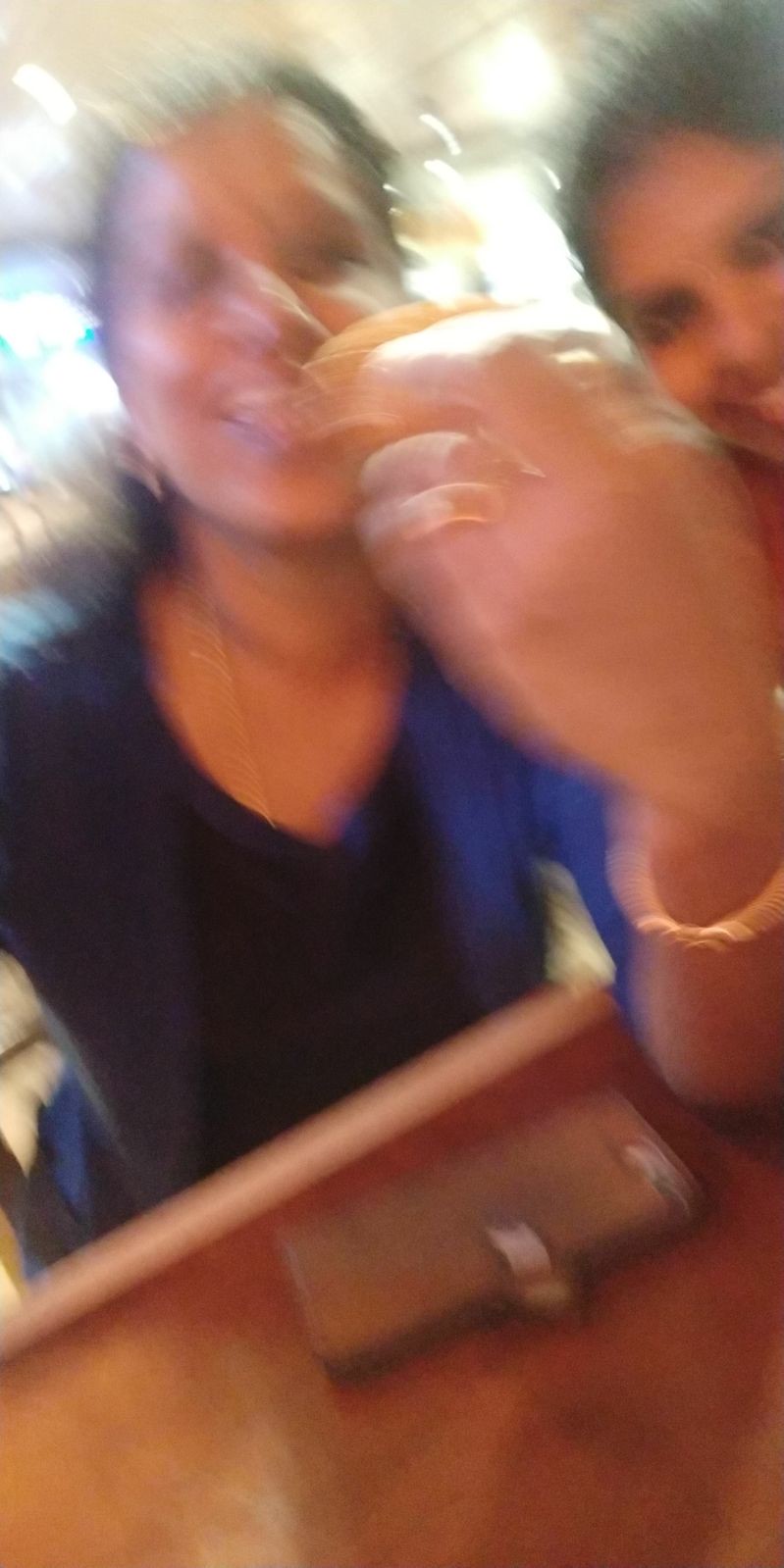This is a color photograph presenting a close-up view of two women with medium skin tones, both smiling. The image is fairly blurred, making it challenging to discern intricate details. The more prominent woman is fully visible, adorned with a blue necklace and dressed in a dark blue top with sleeves reaching at least to her elbows. She also sports a gold bracelet or a watch on her left wrist, which is raised towards the viewer and appears blurred. 

In front of her is a golden-toned wooden table. Positioned on the table is a rectangular, brown leather item, which could be either a wallet or a phone case featuring a latch across its middle. The other woman's face is partially visible to the right of the first woman. The background includes softly glowing lights; bluish on the left and yellow-toned in the space between the two women, adding a warm atmosphere to the scene.